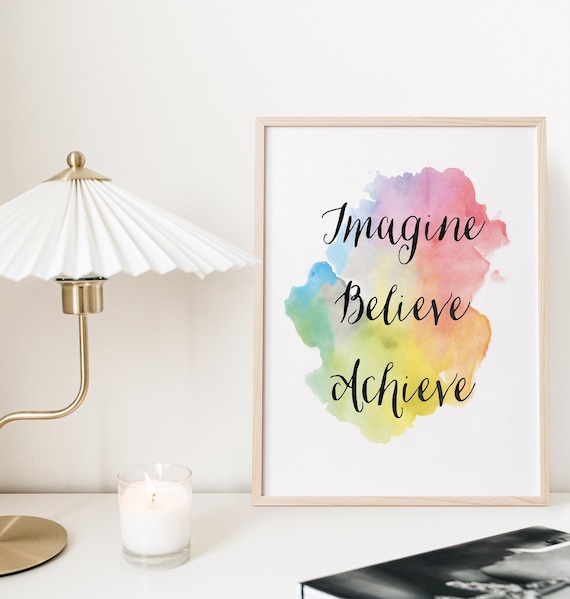The photograph depicts an interior scene centered on a neatly arranged desk against a cream-colored wall. Dominating the left side, there is an elegant bronze-colored lamp with a white lampshade that flares outwards from the base. The base of the lamp is intricately designed, featuring a loop that rises to support the light bulb and culminating in a small bronze globe at the top. 

Next to the lamp, a small clear glass holds a lit white candle, adding a warm, soft glow to the scene. Adjacent to the candle, a light wooden frame encases a motivational plaque. The plaque displays the words "Imagine, Believe, Achieve" in black script, set against a vibrant, multicolored background resembling an oil painting with hues of pink, blue, yellow, orange, and green blending together in a cloud-like formation. 

In the lower right corner of the image, partly jutting out from the desk, is a closed book with a black and white cover that appears to feature a woman's face.